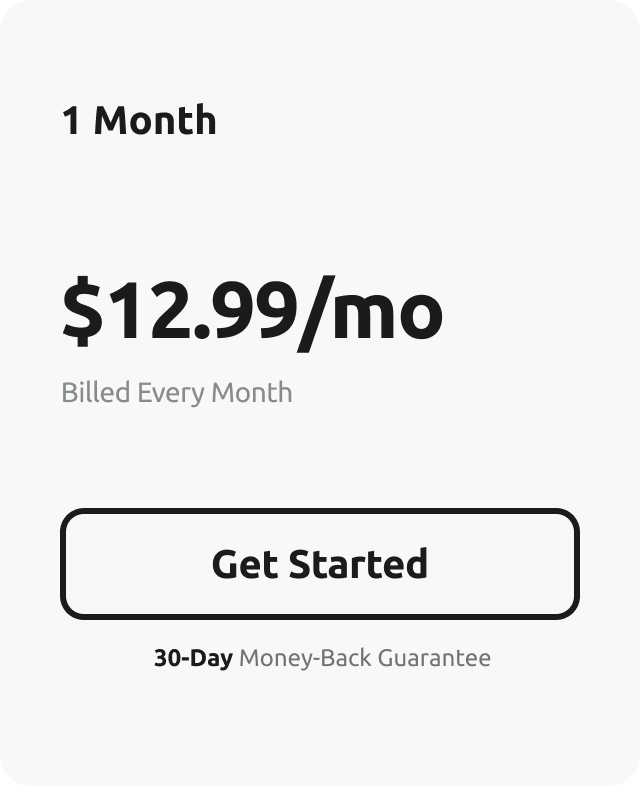The image is a screenshot of a subscription pricing page with a minimalist design featuring a light gray to white gradient background. At the top, the text "One Month" is displayed, with "Month" abbreviated to "M-O." The "O" is followed by a slash, and the price "$12.99 per month" is prominently featured in larger text.

Below the price, the text "Billed Every Month" is shown in smaller, darker gray font with the initials B, E, and M capitalized. 

Further down, a rectangular box outlined in black contains the call-to-action text "Get Started," with the "G" and "S" capitalized.

At the bottom of the screenshot, the text "30-Day Money-Back Guarantee" is displayed in a slightly darker gray font. The "D" in "Day" and the initials "M," "B," and "G" in "Money-Back Guarantee" are capitalized, with a dash between "Money" and "Back."

All the text, including "$12.99 per month," "One Month," "Billed Every Month," "Get Started," and "30-Day Money-Back Guarantee," uses a consistent font style throughout the screenshot, suggesting a cohesive and professional presentation. This screenshot appears to be from a billing plan or subscription page.